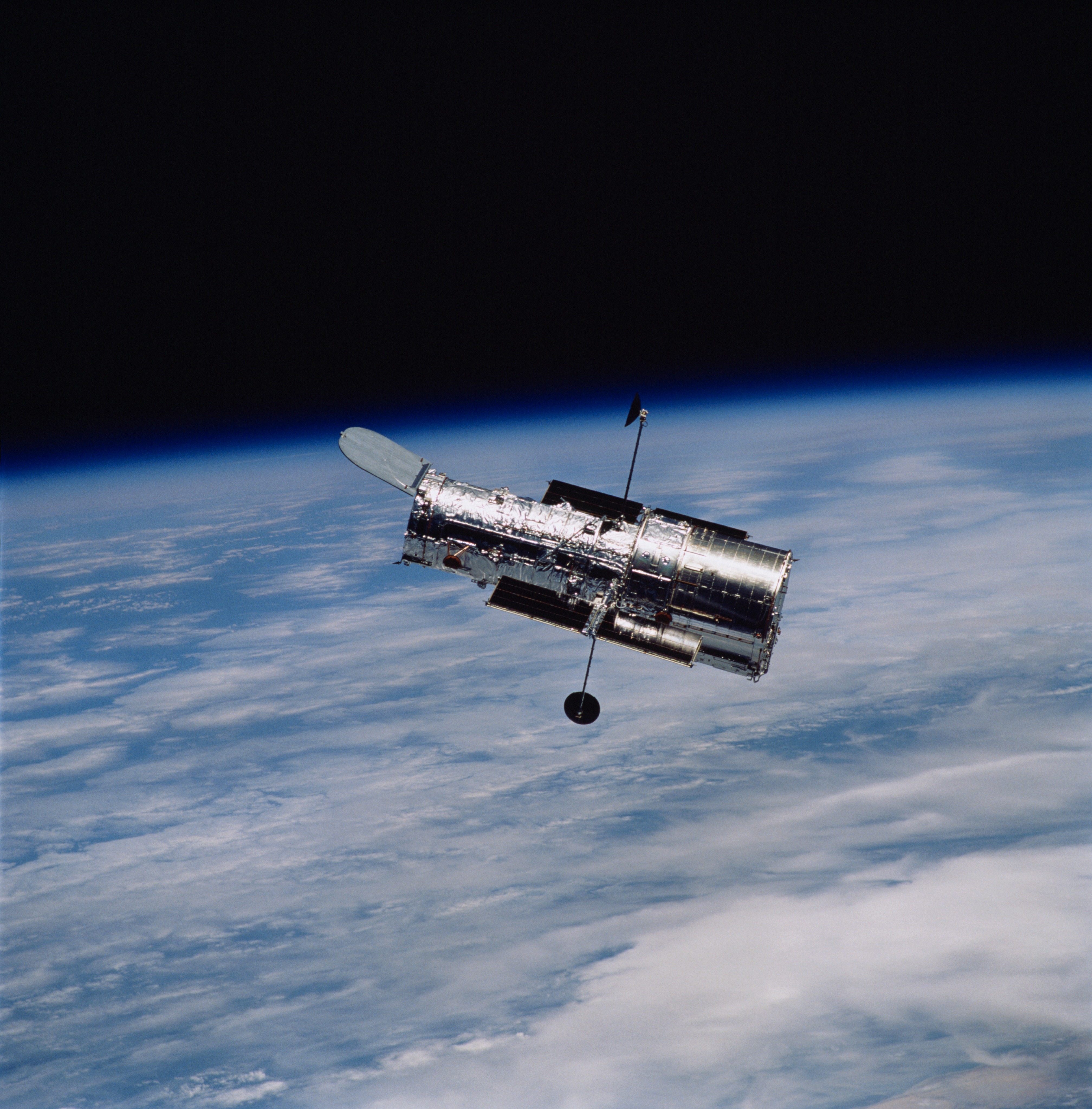In this detailed image, a shiny, silver satellite is floating in the blackness of space just above Earth. The satellite appears to be constructed with tin-like materials and features a wrapping that resembles aluminum foil on its left side. Two circular sensors or satellite dishes are clearly visible, supported by black metal rods. There is also an open flap on the left side of the satellite. Below the hovering satellite, Earth is partially visible, displaying an expanse of clouds, blue skies, and portions of the ocean. Additionally, a stretch of land, including a beach, can be seen in the bottom right corner. The satellite seems to be monitoring or studying something, although its exact purpose is unclear.